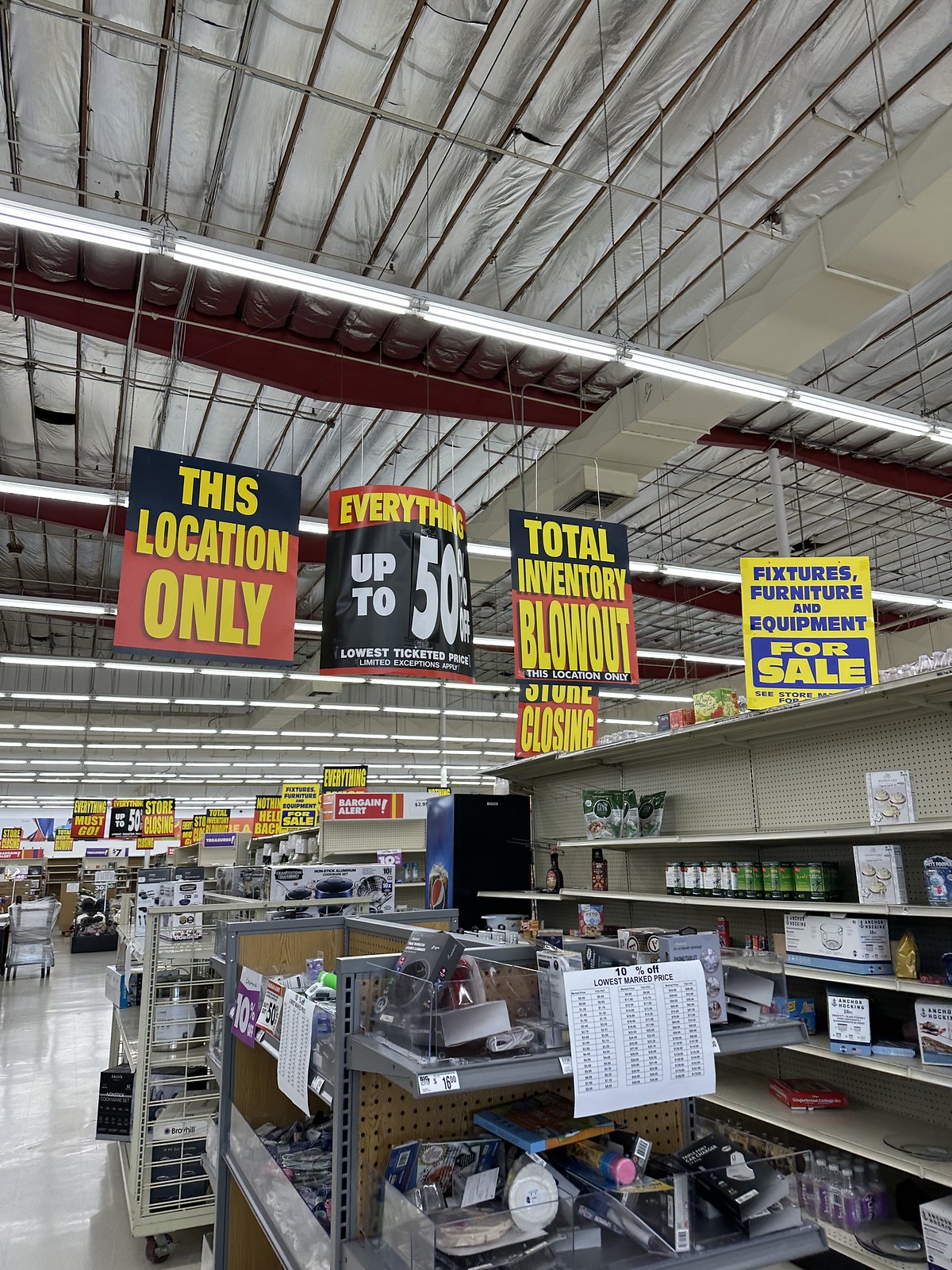In the photograph, a man is standing inside a large store aisle surrounded by various shelves filled with food products, jars, and small cardboard boxes, though the labels are too distant to read clearly. Closer to the foreground, random and seemingly disorganized racks and trays of miscellaneous physical products are scattered about. The high ceiling of the store is lined with long lights running the length of the area, while a network of rafters is visible above. Numerous colorful signs dangle from wires overhead, announcing a major clearance event. The prominent signs are black on top with red bottoms, featuring bold yellow and white lettering, proclaiming offers like "this location only," "everything up to 50% off," and "total inventory blowout." Beneath one of these signs, another one reads "store closing." Additionally, a yellow sign with blue writing advertises the sale of fixtures, furniture, and equipment, enhancing the sense of a closing-down sale with significant markdowns on all items.